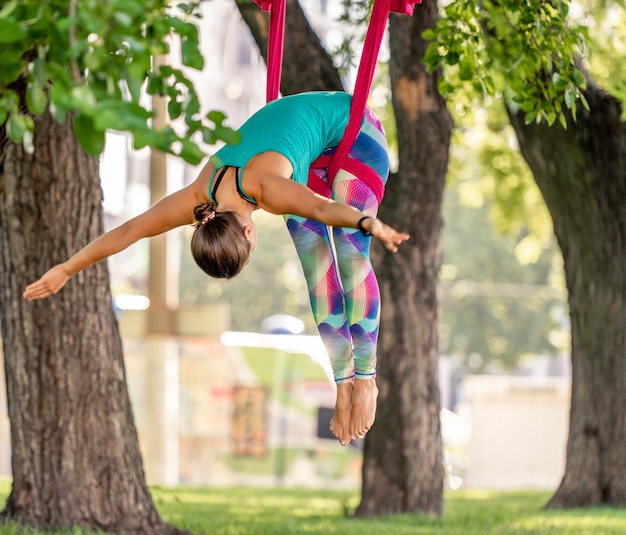The image captures an aerial performer suspended gracefully from a burgundy ribbon amidst a forested backdrop. The scene features several thick tree trunks with lush green leaves, but the background is slightly out of focus, enhancing the ethereal quality of the composition. The performer, resembling a circus aerialist, is dressed in a light blue tank top and colorful leggings streaked with shades of pink, blue, light blue, purple, yellow, and green. Her brown hair is styled in a low bun, and her head is bowed down as she hangs elegantly from the ribbon. Her arms are spread wide open, and her legs are securely strapped to the ribbon, with her toes pointed in an artistic pose. The overall composition blends the natural beauty of the forest with the artistry of aerial performance.